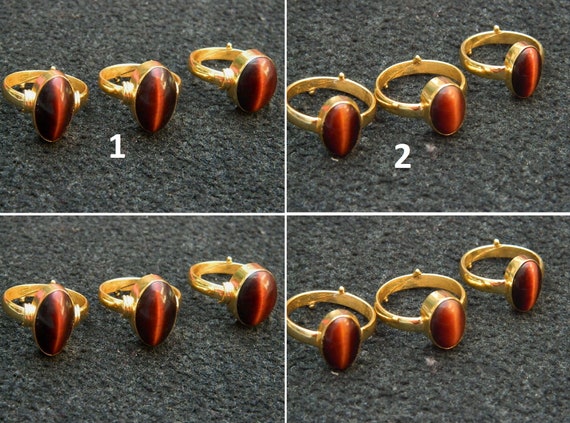The set of images consists of four closely related photographs arranged in a grid with two images on the top row and two on the bottom row, separated by thin white lines that form a crosshair-like pattern. Each photograph showcases three golden rings, each adorned with a reddish-brown stone that features a striking vertical light-red stripe down the center.

In the top-left image, labeled with the number "1," the rings are oriented to highlight this vertical stripe against their rich golden bands. The top-right image, labeled with the number "2," shows a similar perspective but with a slight variation in the ring's angle which makes the central light-red stripe appear more pronounced and brighter.

The bottom row comprises two more images that seemingly replicate the top-row perspectives but without any number labels. The bottom-left image mirrors the view of the top-left, where the rings are displayed with the vertical stripe visible yet more subdued. In contrast, the bottom-right image mirrors the top-right image, spotlighting a much brighter central stripe that dominates each stone's appearance.

The stones in the rings, possibly resembling tiger's eye, exhibit a captivating light-red starburst stripe which shifts in intensity based on the photographic angle, providing a dynamic visual experience across the four images.